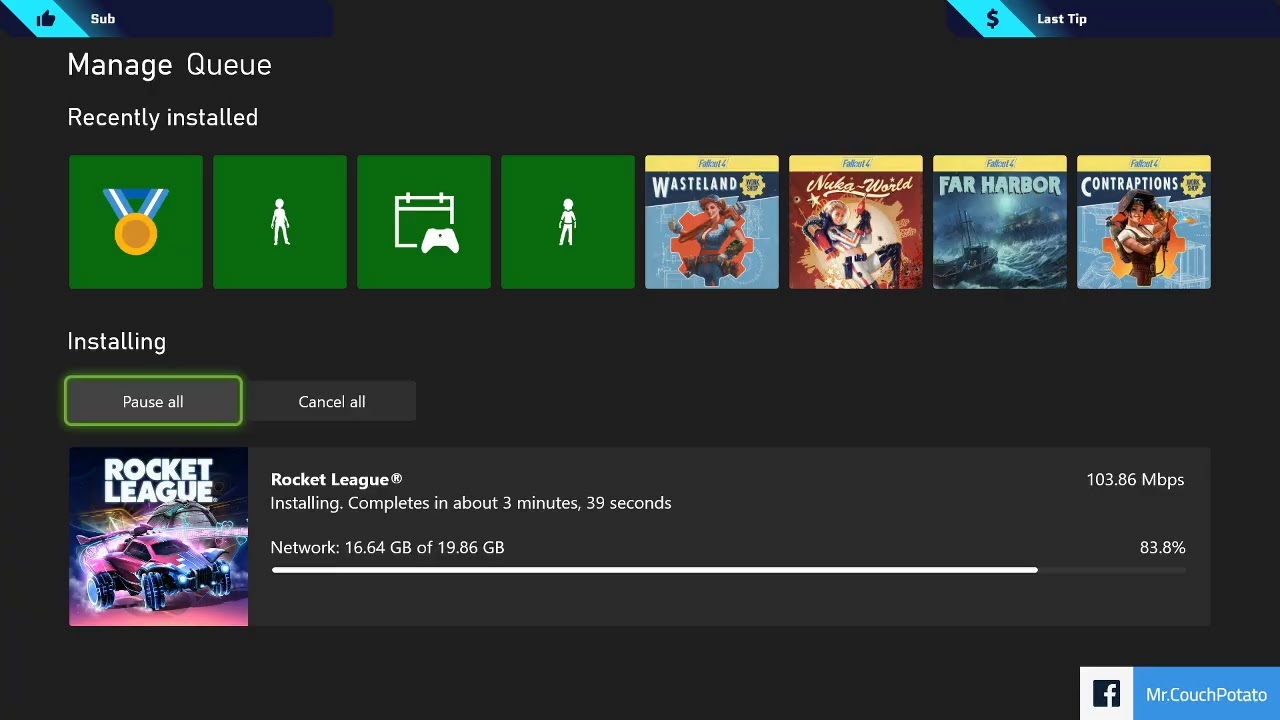This image portrays a section of a game website, likely part of a game management app interface. At the top of the screen, there is a label that says "Sub." On the left side of the interface, there is a section labeled "Last Tip," followed by another section marked "Manage Queue." Below that, there is an area titled "Recently Installed."

On the right side of the screen, various icons and images are visible. Notable among these is a small icon depicting a woman in a white outline on a green background, followed by the outlines of a calendar and a game controller. Additionally, an icon showing the outline of a man is visible.

Adjacent to these icons are two illustrated posters for the game "Fallout 4," featuring women in a 1950s pin-up style. Below these posters, there is another illustration related to "supported water," followed by another pin-up style image of a woman.

At the bottom of the image, a status update indicates that "Rocket League" is currently being installed.